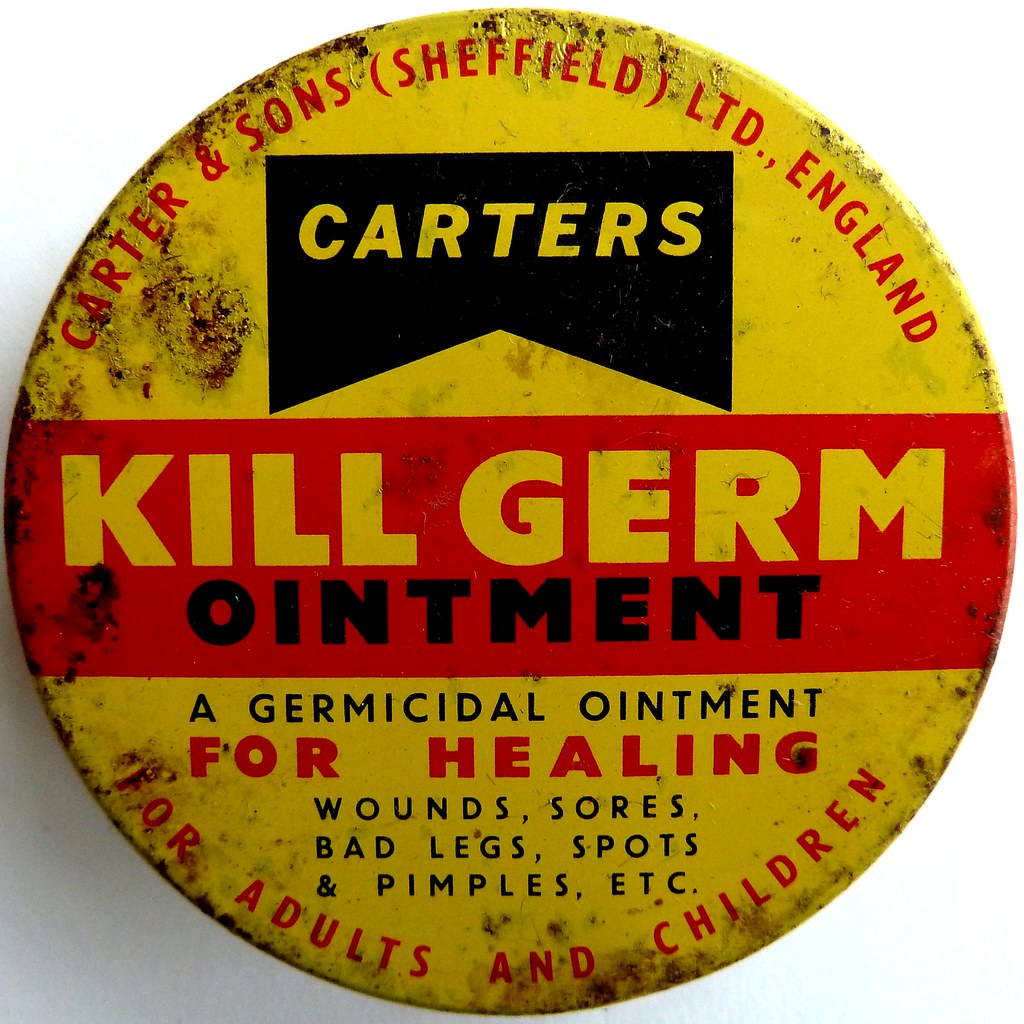The image is a top view of a very old, circular lid of a can of ointment, showing significant signs of wear and rust. The lid is predominantly yellow with areas where the paint has come off, exposing rusting spots and a metal base. At the top edge, in red arched text, it reads "Carter and Sons Sheffield Limited England." Beneath this, there is a black ribbon logo with the word "Carter's" in yellow letters. Across the middle of the lid, there is a prominent red banner with the text "KILL GERM" in yellow capital letters, followed by the word "OINTMENT" in black. Below this banner, it states in black text, "A germicidal ointment for healing wounds, sores, bad legs, spots, and pimples, etc." Finally, at the bottom edge in red curved text, it reads, "For adults and children." The lid is heavily damaged, reflecting its age and prolonged use.